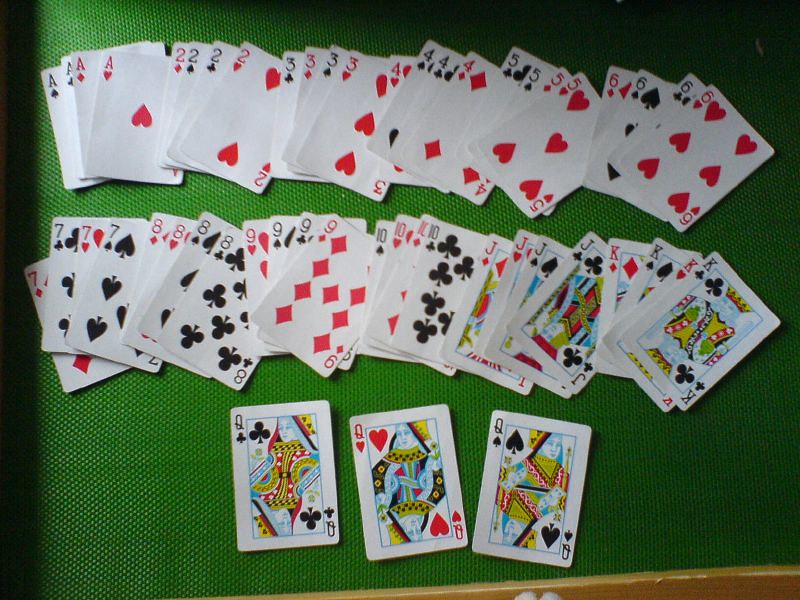An overhead photograph captures an intricately woven green fabric with a rough texture, possibly the surface of a playing table. The composition also includes an edge of light-colored wood at the bottom, suggesting the table's border. On the left-hand side of the photo, a significant black stripe, likely a shadow, adds contrast to the scene.

Spread meticulously across the green fabric are face-up playing cards, organized in an orderly fashion. At the top left, all four aces are neatly aligned: spades, clubs, diamonds, and hearts. Directly beneath them, the twos are placed in a similar manner. This pattern continues with the threes, fours, and fives arranged sequentially and shifted to the right in rows. Moving further to the right, the order continues with the sixes.

A new row features sevens, followed by the eights, nines, and jacks. To the right of these cards, fully visible are all the kings. However, one card is conspicuously missing; while the bottom row displays the queens of clubs, hearts, and spades, the queen of diamonds is absent, leaving an incomplete deck.